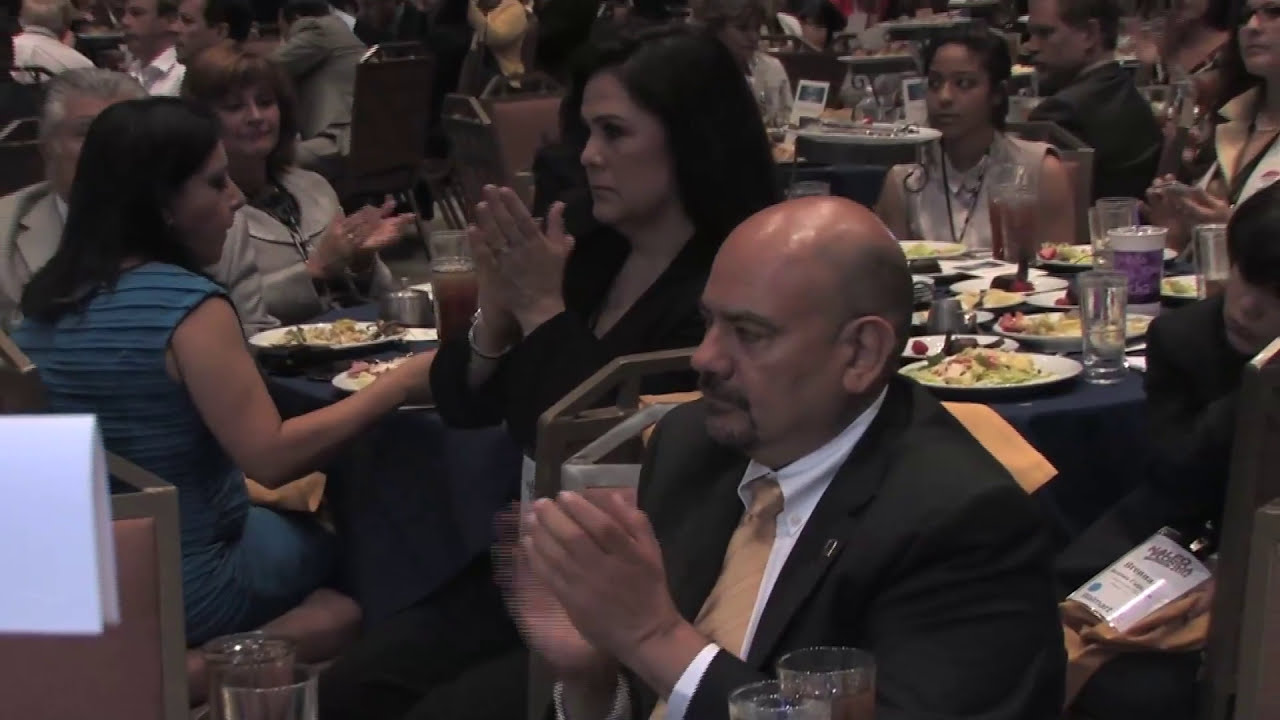This photograph depicts a formal dinner or banquet scene with a group of people seated around round tables adorned with blue tablecloths, food, and glasses with various beverages. The crowd, primarily adults with a few young children, seems to be listening to a guest speaker, as many are clapping despite their generally stern expressions. Central in the foreground, a balding man with a mustache and goatee is dressed in a black suit with a white shirt and a yellow tie, claps with four glasses placed on the table around him. Behind him, a young boy, clad in a black suit jacket and holding a white pass on a chain, leans wearily against the back of a chair. Nearby, a woman with long, dark hair wearing a black dress sits next to another woman in a sleeveless blue-and-black striped dress who is eating. The overall ambiance is somewhat muted with less vibrant colors, suggesting subdued lighting.